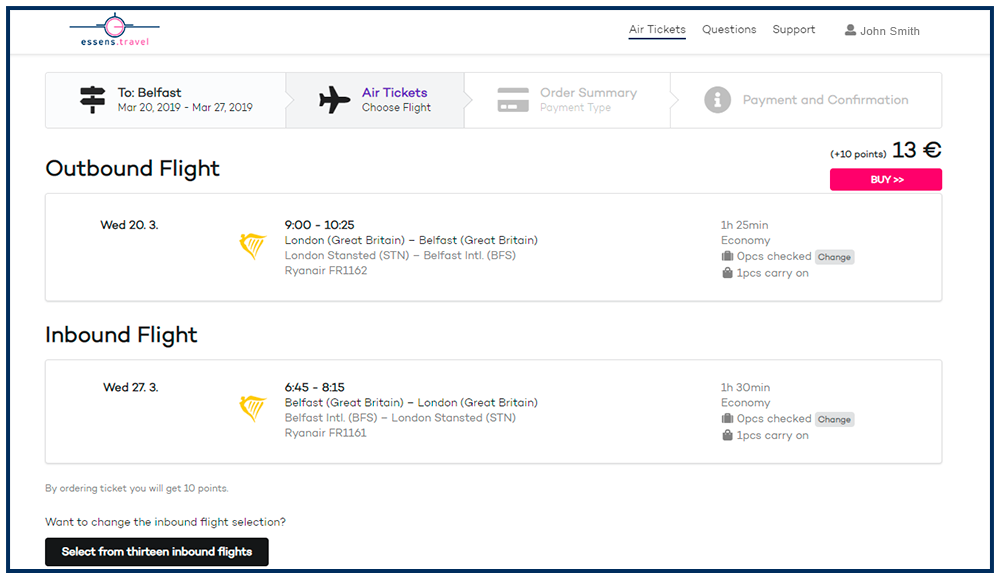The image displays a screenshot of a desktop computer screen showcasing the Center Travel website, set against a white background. The interface is encased in a dark blue rectangular border. At the top, the focal point is the logo, which features a stylized 'C' in white against a blue and pink backdrop. The logo text reads "Center" in blue and "Travel" in pink.

To the right of the logo, on the same line, there are menu options: "Add Tickets" (underlined), "Questions," "Support," and a profile area labeled "John Smith," all written in gray text. 

Below the header, there are travel details: 
- From: Belfast
- Dates: March 20, 2019, to March 27, 2019

Further down, the interface allows users to select their flights with sections for "Choose Flights," "Summary," and "Payments and Confirmation." The "Outbound Flights" indicates departure details, including the ticket price of 13 pounds. Near this information, there is a prominently displayed pink button with white arrows and the word "Buy" indicating the action to finalize the ticket purchase.